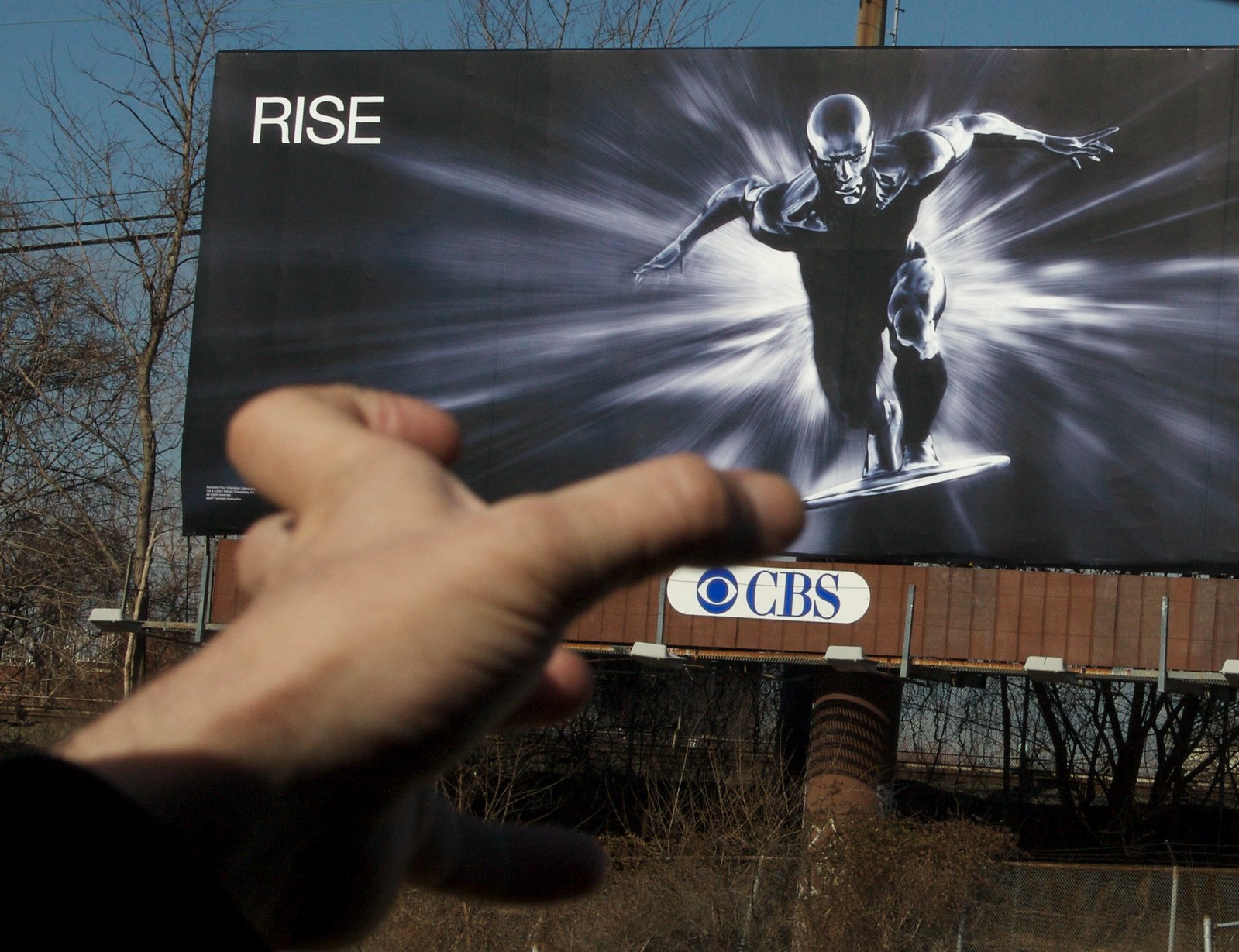In the image, there is a colossal billboard featuring a dynamic superhero character. The top left corner of the billboard prominently displays the word "RISE" in large, bold white letters. The superhero is depicted in a powerful take-off pose, as if caught in mid-motion, racing forward with an intense burst of speed. The background accentuates this sense of rapid movement with vibrant, blurred lines, enhancing the feeling that the character is set to shoot through the air at high velocity. The billboard is situated in a secluded area surrounded by dense trees and branches, making the enormous signage stand out even more amidst the natural setting. Below the billboard, the CBS logo is clearly visible, lending a clue to the network associated with the advertisement.